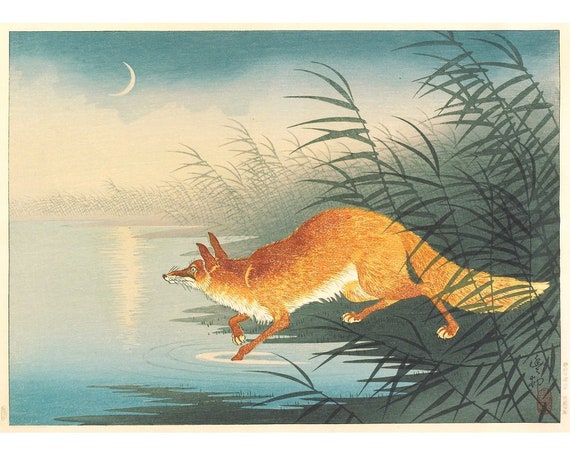This painting depicts a fox with an orange-brown coat and a white chest, cautiously extending its front paws into a body of water, likely a pond, situated on the left side of the image. The fox, viewed in side profile, appears to be intently looking or smelling for something along the water's edge. It has a long, bushy tail and darker fur near its ears and feet. The background features a sky with a small crescent moon casting its gentle light over the scene, complemented by patches of white and blue. The right side of the composition is filled with grayish-green grass and tall green bulrushes lining the bank. The atmosphere is enriched by some visible fog, adding a sense of mystery to the tranquil setting.